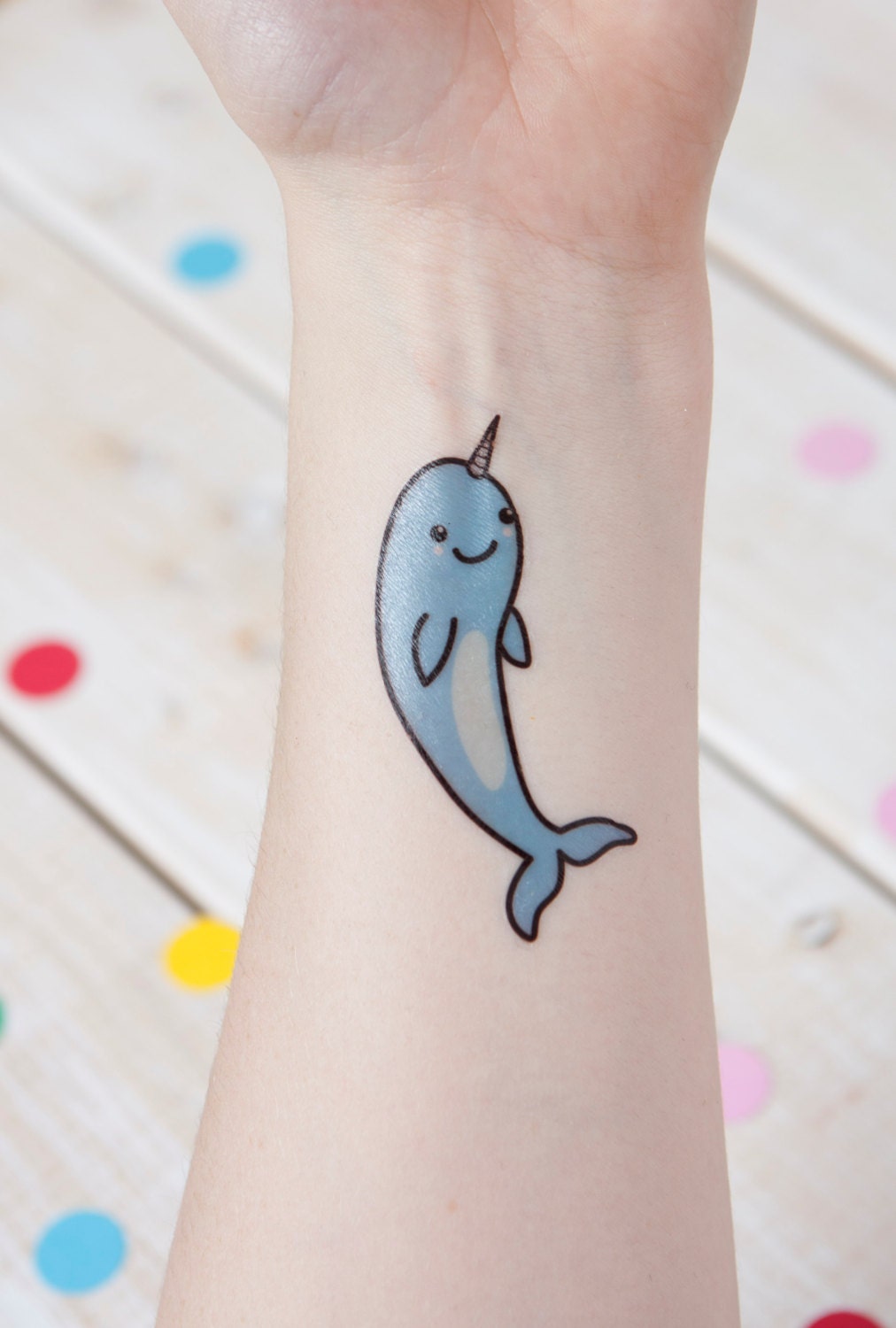This is a color photograph of the left forearm of a light-skinned individual, prominently displaying a whimsical, temporary tattoo. The tattoo depicts a cute, childlike narwhal in a light baby blue hue with a white belly, outlined in black. The narwhal has a friendly smile, two black eyes, two fins, a tail, and a distinctive, black spiky horn on its forehead, somewhat akin to a unicorn's. The background features wooden planks, possibly the surface of a picnic table, adorned with sporadic, brightly-colored polka dots in shades of red, yellow, light blue, pink, and another blue, adding a playful element to the scene.